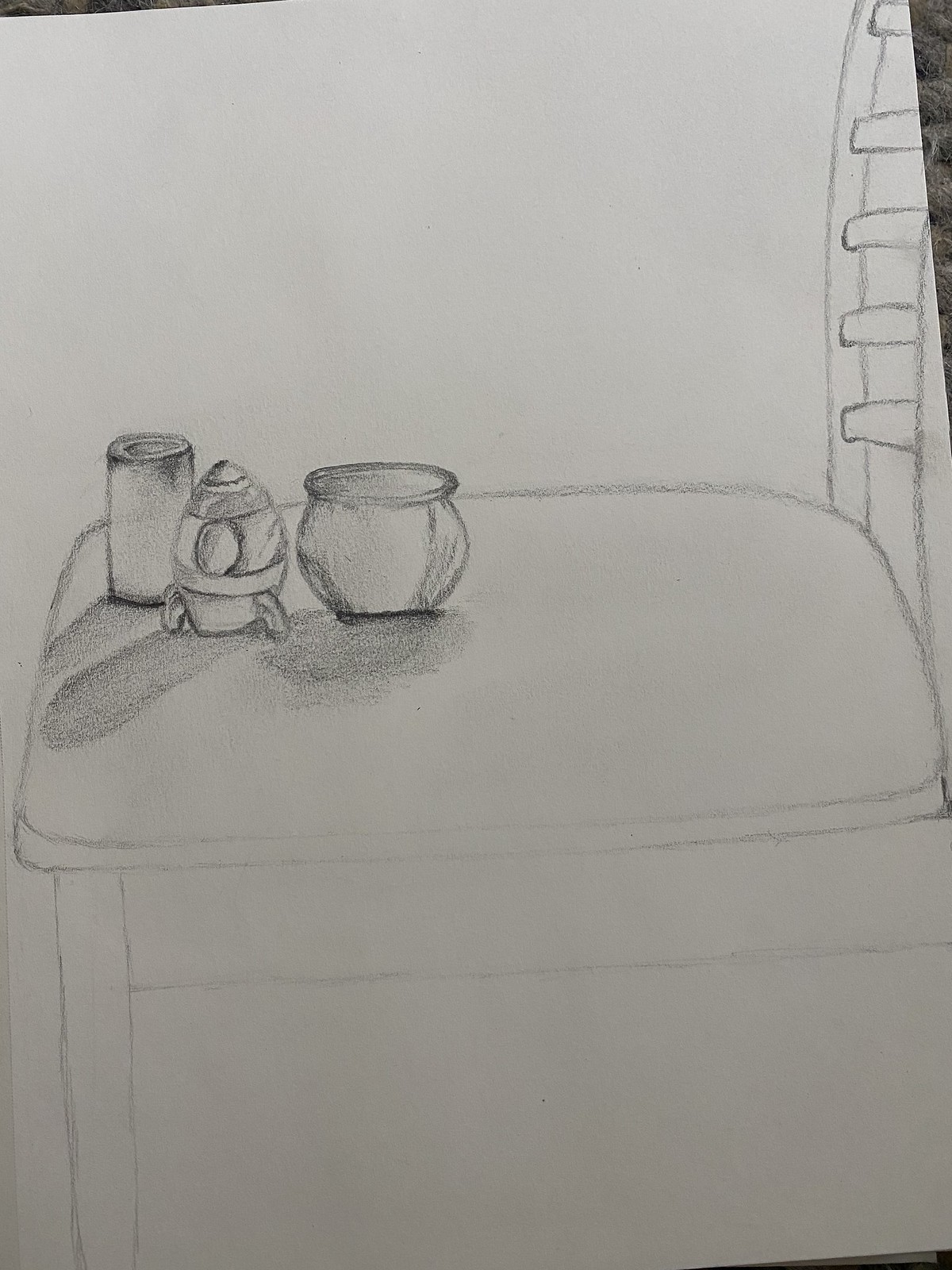A detailed photograph captures a pencil sketch on a white piece of paper. The sketch, rendered in a dark black pencil, depicts a rough outline of a wooden chair. The chair, detailed with visible legs and a seating surface, features a backrest composed of several horizontally aligned wooden posts. Atop the chair's seat are three distinct objects: a small pot, a cylindrical object, and what appears to be a miniature spaceship. The edges of the paper are visible, revealing it resting on a table that seems to be made of gray stone.